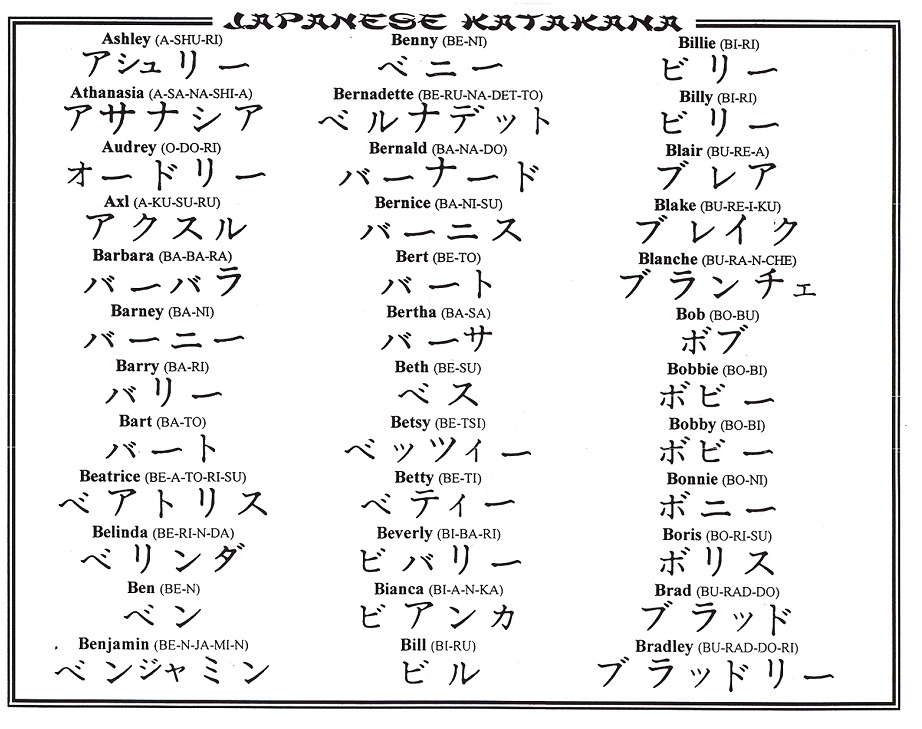This detailed poster, titled "Japanese Katakana" at the top in bold, showcases a conversion of American male and female names into Japanese Katakana script. The white background with black print features three columns, each containing 12 names, resulting in a total of 36 names. Starting with "Ashley" and ending with "Bradley," each English name is followed by its phonetic breakdown in parentheses and the corresponding Katakana characters. For instance, "Ashley" is rendered as "Ashuri," "Benny" as "Bini," and "Billy" as "Bairai." The poster provides a comprehensive guide to understanding how these names are pronounced and written in Japanese, making it both educational and interesting.